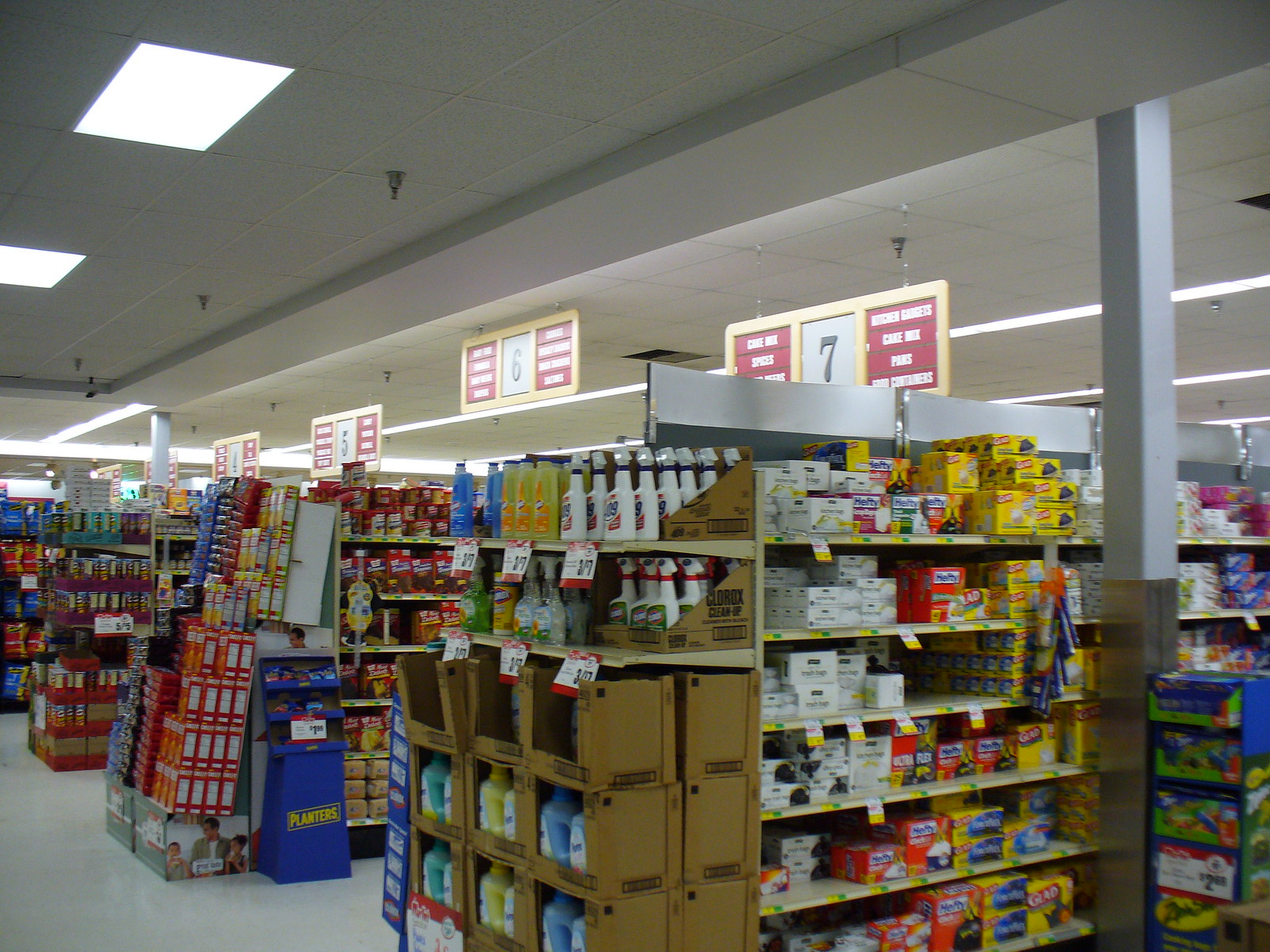This detailed photograph captures the interior of a grocery store taken from the end of one aisle, offering a clear view down several adjacent aisles numbered with signs hanging from the ceiling. The nearest visible aisle is marked as Aisle 7 with a black-on-white sign, flanked by red labels detailing the contents, including kitchen gadgets, cake mixes, pies, pans, and spices. Beyond Aisle 7, you can see the numbers for Aisles 6, 5, 4, and likely in the distance, Aisles 3, 2, and 1. 

The white ceiling is dotted with silver fire sprinklers and rectangular fluorescent lights embedded in the panels. The shelves visible within the image primarily stock cleaning and kitchen products. On Aisle 7, there are garbage bags, including brightly colored boxes of Hefty bags and Ziploc boxes. Additionally, you can spot a variety of cleaning products such as 409 cleaner in blue and white bottles, yellow bottles of unspecified cleaner, Clorox cleaner in white bottles with green labels, and Clorox wipes with yellow labels. There are clear bottles with multi-colored labels and a squirt bottle with green fluid. At the base are open boxes containing fabric softeners in light blue, yellow, and pale green bottles.

Adjacent to this, the next aisle has canned frosting in red cans and cake mixes in red boxes. Toward the end of this aisle is a blue display featuring Planters nuts and an assortment of snack crackers like Cheez-Its in red boxes, interspersed with yellow and blue packaging for various snacks. The floor is finished with linoleum, and two visible pillars add to the store's structural details.